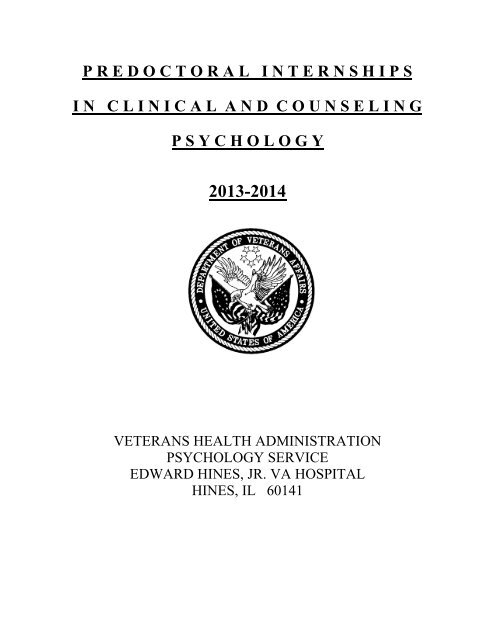Screenshot of a Document Cover Page: 

The cover page is white with black text and features an official symbol at the center. At the very top of the page, the title reads in all caps and underlined, "PRE-DOCTORAL INTERNSHIPS IN CLINICAL AND COUNSELING PSYCHOLOGY, 2013-2014." 

The central emblem is encased within a circle. At the top arc of the circle, written in white letters on a black background, is "Department of Veterans Affairs." The bottom arc of the circle reads "United States of America." 

The emblem itself features a bird with outstretched wings, positioned in front of a sun. Flanking the bird are two flags, adding to the emblem's patriotic imagery.

At the bottom of the cover page, in all caps, it states: "VETERANS HEALTH ADMINISTRATION PSYCHOLOGY SERVICE, EDWARD HINES JR. VA HOSPITAL, HINES, IL 60141."